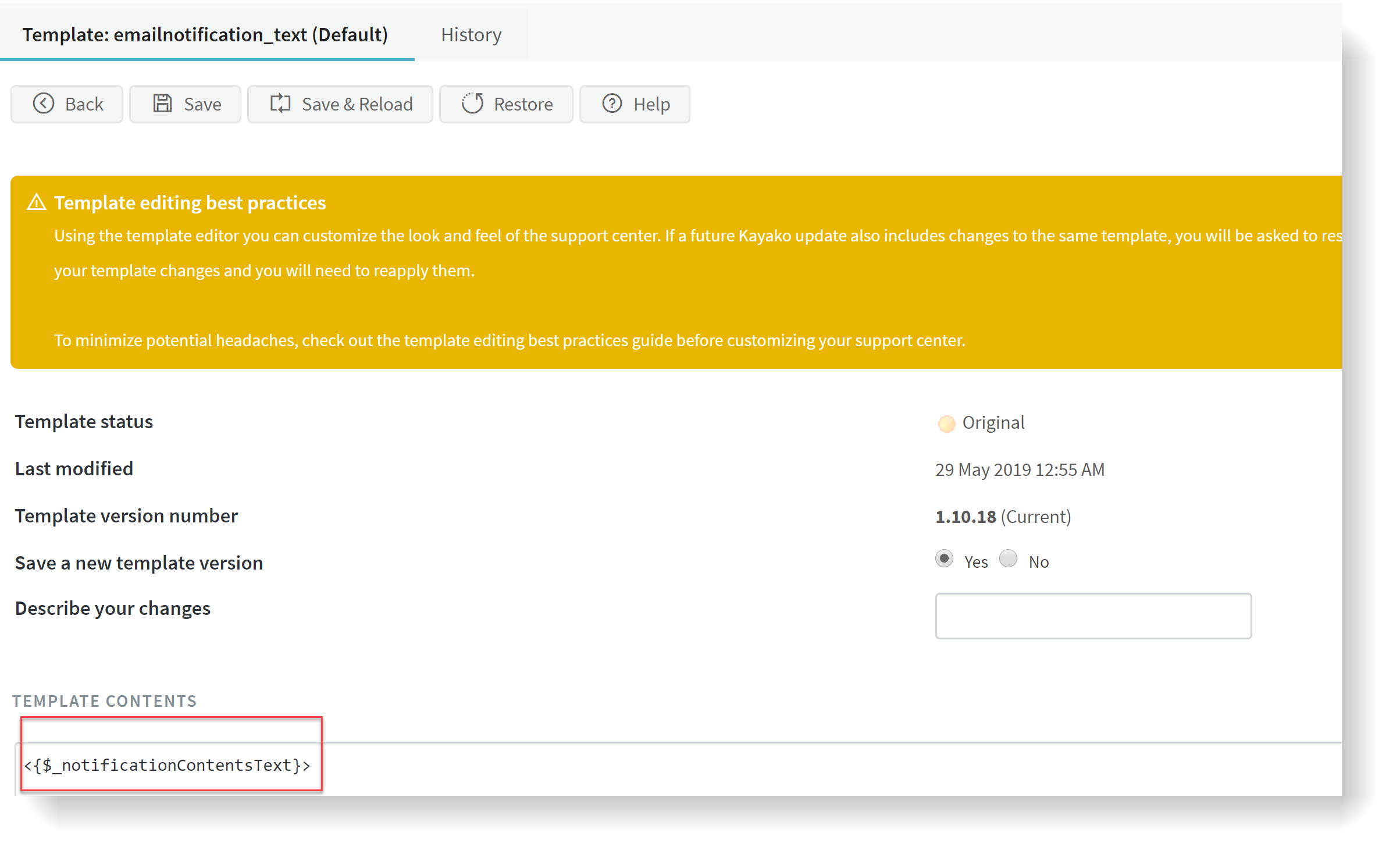The image displays a screenshot of a template editing interface for an email notification system. In the top left corner, "Template Email Notification_Text_Text Default_History" is underlined in blue. Directly below this title are five functional tabs labeled: Back, Save, Save and Reload, Restore, and Help.

On the left side, beneath the tabs, there's a highlighted notice with an orange background and white text. This notice reads:

"Template Editing Best Practices

Using the template editor, you can customize the look and feel for the support center. If a future Kayako update includes changes to the same template, you will be asked to restore your template changes and reapply them. To minimize potential headaches, check out the template editing best practices guide before customizing your support center."

Beneath the notice, the background shifts to white. On the left, it states "Template Status," while on the right, it details: 
"Original Last Modified: 28 May 2019, 12:55 AM
Template Version Number: 1.1.0.18
Current Save a New Template Version: Yes or No (Yes is selected)"

At the bottom left corner, there’s a section outlined in a red card indicating "Describe Your Changes: Template Content, Notification Content."